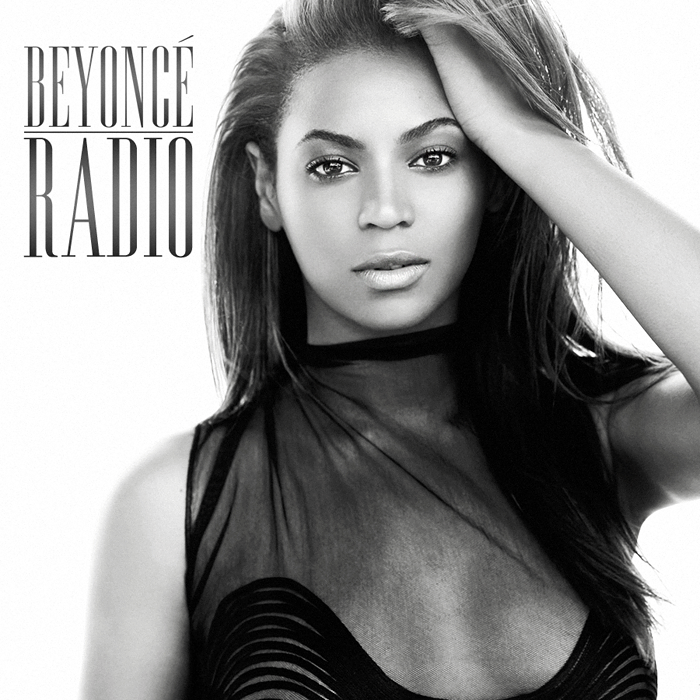The image features a black and white photograph of Beyoncé Knowles, formerly of Destiny's Child, on what appears to be the cover for a single record titled "Beyoncé Radio." In the upper left-hand corner, the title "BEYONCÉ RADIO" is prominently displayed in capital black letters, with "BEYONCÉ" positioned above "RADIO." The background is stark white, which accentuates Beyoncé's striking presence. Beyoncé, with her café au lait-colored skin, is pictured with her left hand running through her light-colored, shoulder-length hair, while her right hand remains out of view. Her eyes, described as sparkly yet dark, peer directly into the camera beneath her arched eyebrows, and her lips are closed without revealing her teeth. She wears a glamorous black outfit that combines a sheer, mesh top with a more opaque bodice below, creating a sophisticated yet edgy look. The overall image is meticulously styled, highlighting her elegance and star power, making it a captivating promotional cover for a single record or radio show.